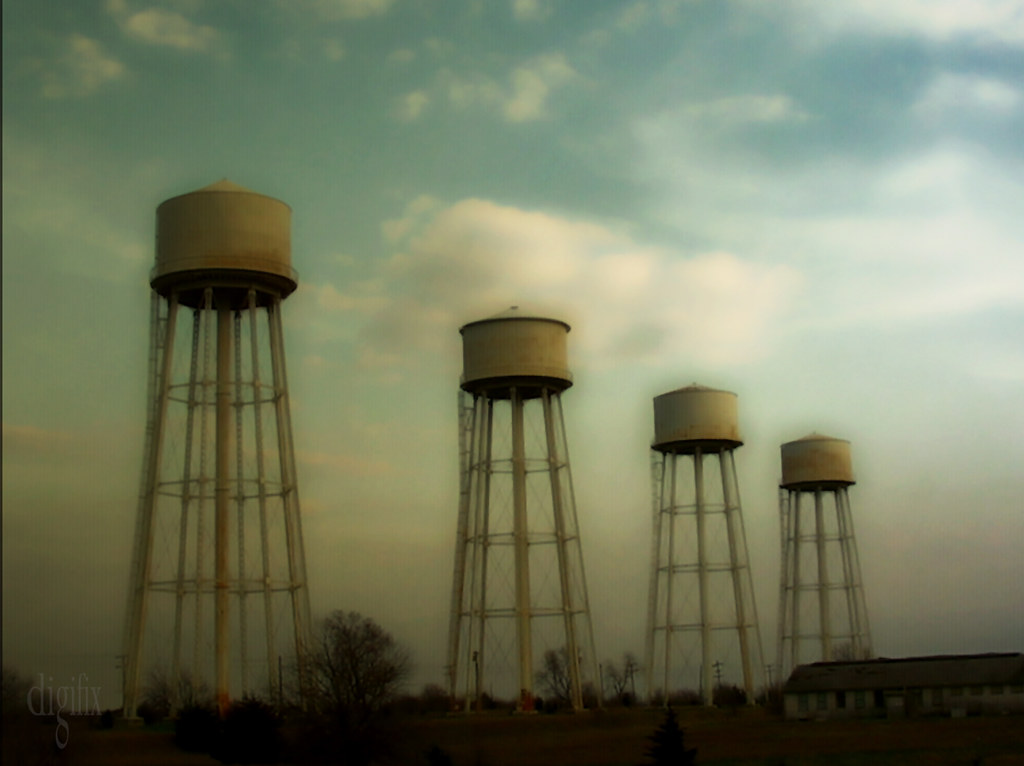The image depicts four water towers, their cylindrical tanks supported by triangular, cylindrical stands with numerous pillars for stability. Light brown in color, both the tanks and their structures feature central pipes descending downwards and staircases for access. Positioned in a row, the towers appear to vary in height due to perspective, progressively shrinking from left to right. Above, the sky is a slightly dim blue with scattered clouds, giving the scene an evening ambiance. A house with brown roofing and cream-white walls sits in the bottom right corner, accompanied by a few trees that reach about a fifth of the towers' height, reinforcing their impressive stature. The overall scene, possibly a painting, carries a somewhat dark, melancholic tone. In the bottom left corner, the word "DigiFix" is written in white.